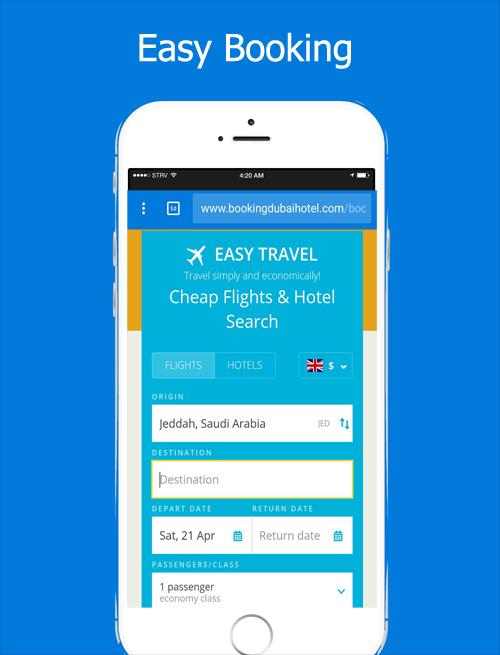In this image, we see a screenshot displayed against a solid blue background. At the top of the image, bold white text reads "Easy Booking." Below this heading, there is a photo of a white Apple iPhone. The left side of the phone features two similarly sized buttons with a smaller white button positioned above them. On the right side, there is a silver button. The iPhone screen displays various status indicators at the top: four out of five circles are lit up, indicating signal strength, the Wi-Fi icon is visible, the time reads 4:20 a.m., and the battery appears to be full.

The main part of the iPhone screen features a blue background with a search or address bar that reads "www.bookingdubihotel.com." Below this bar, there is an icon of a white airplane accompanied by text on its right that states "Easy Travel.” Additional promotional text underneath reads, "Travel simply and economically. Cheap flights and hotel search."